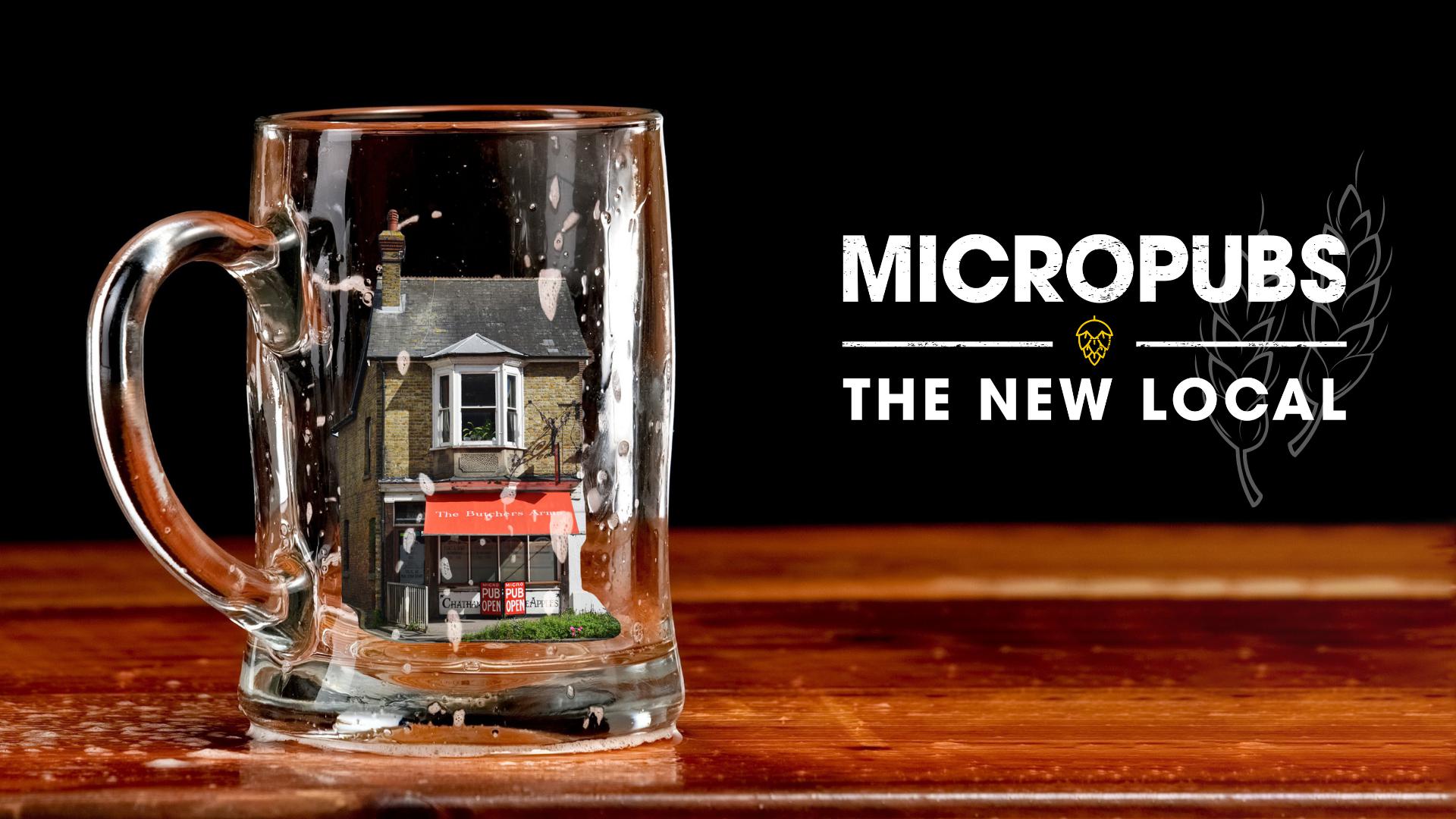A detailed photograph showcases an empty pint glass on the left side, resting on a medium-toned wooden bar top with traces of beer foam. The black background contrasts sharply with the reflective surface of the glass, which intriguingly contains the image of a two-story, tan house-turned-pub. This house features a black roof, two chimneys at either end, and a distinctive awning extending over the first story, covering about two-thirds of the width at the front. Below the awning, a red box and a green lawn with a wall leading up to it are visible. On the right of the glass, in capital white letters, the text reads "Micro Pubs" above a golden emblem, framed by two white lines, and below this design, it says "The New Local." This composition creates an engaging and sophisticated business advertisement set against an elegantly dark backdrop.